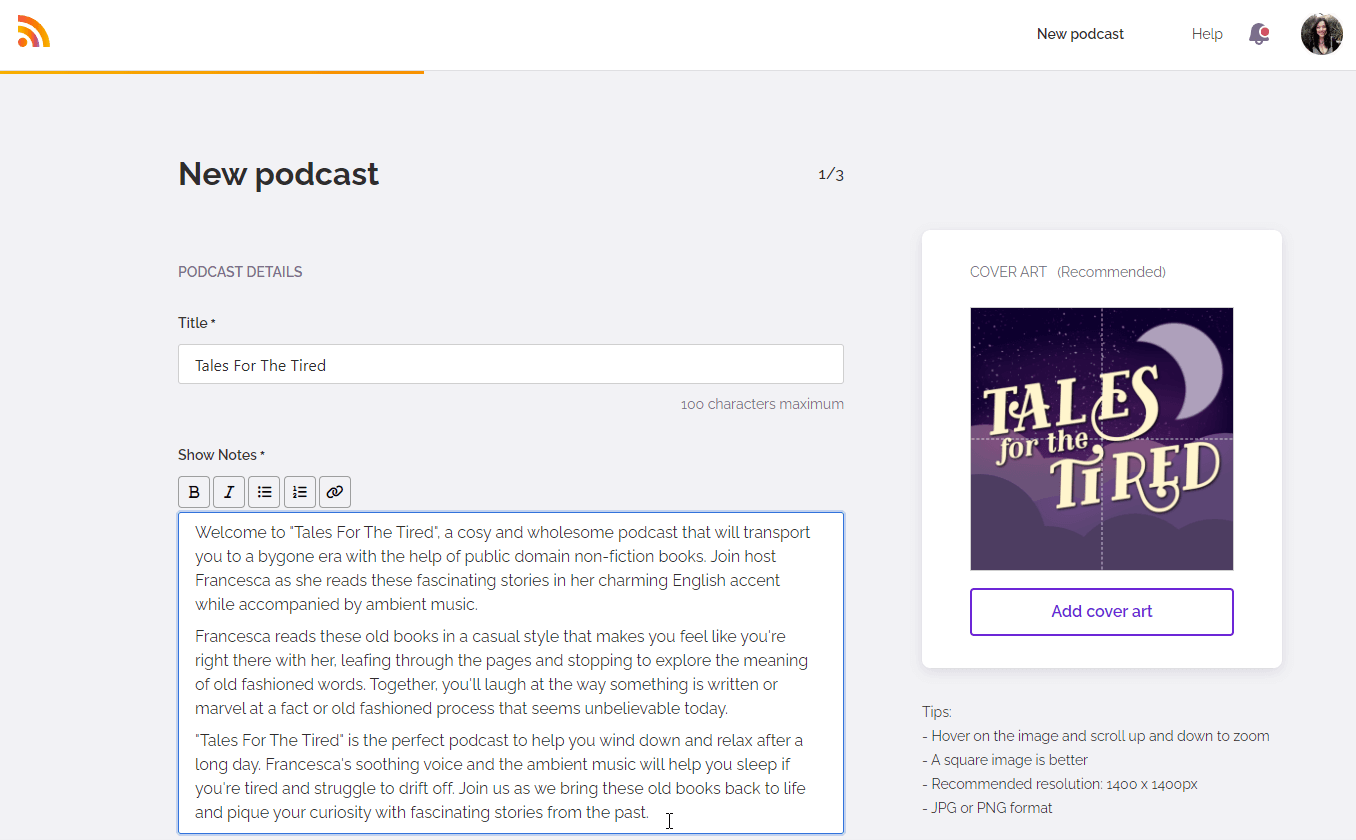**Caption:**

This landscape-oriented screenshot showcases the interface of a podcast application, likely Audible. In the upper left corner, the Audible logo is prominently displayed. The upper right corner features a notification bar with a red dot and what appears to be a female avatar, indicating new podcast help notifications. 

Dominating the top portion of the screen is a bold header in a gray section that reads "New Podcast" with a subtitle showing "1 of 3." Below, the interface splits into two columns. 

On the left column, details are requested for the new podcast. The form fields include:
- **Title**: "Tales for the Tired" (with a minimum character count requirement of 100).
- **Show Notes**: A text area where the introductory text reads, "Welcome to Tales for the Tired, a cozy and wholesome podcast that will transport you to a by-gone era."

Further elaboration explains the podcast’s content, highlighting that "Francesca reads old books in a casual style that immerses listeners as if they were leafing through the pages together, exploring the meanings of old-fashioned words, and laughing or marveling at historical processes."

On the right column, it focuses on the podcast's visual aspects. There is a section for cover art titled "Recommended Tails for the Tired," featuring a placeholder button labeled "Add Cover Art." It provides tips emphasizing the preferred image format (square) and the recommended resolution (JPG or PNG).

Overall, the image comprehensively details the process of submitting a new podcast, especially focusing on content and visual guidelines for "Tales for the Tired."